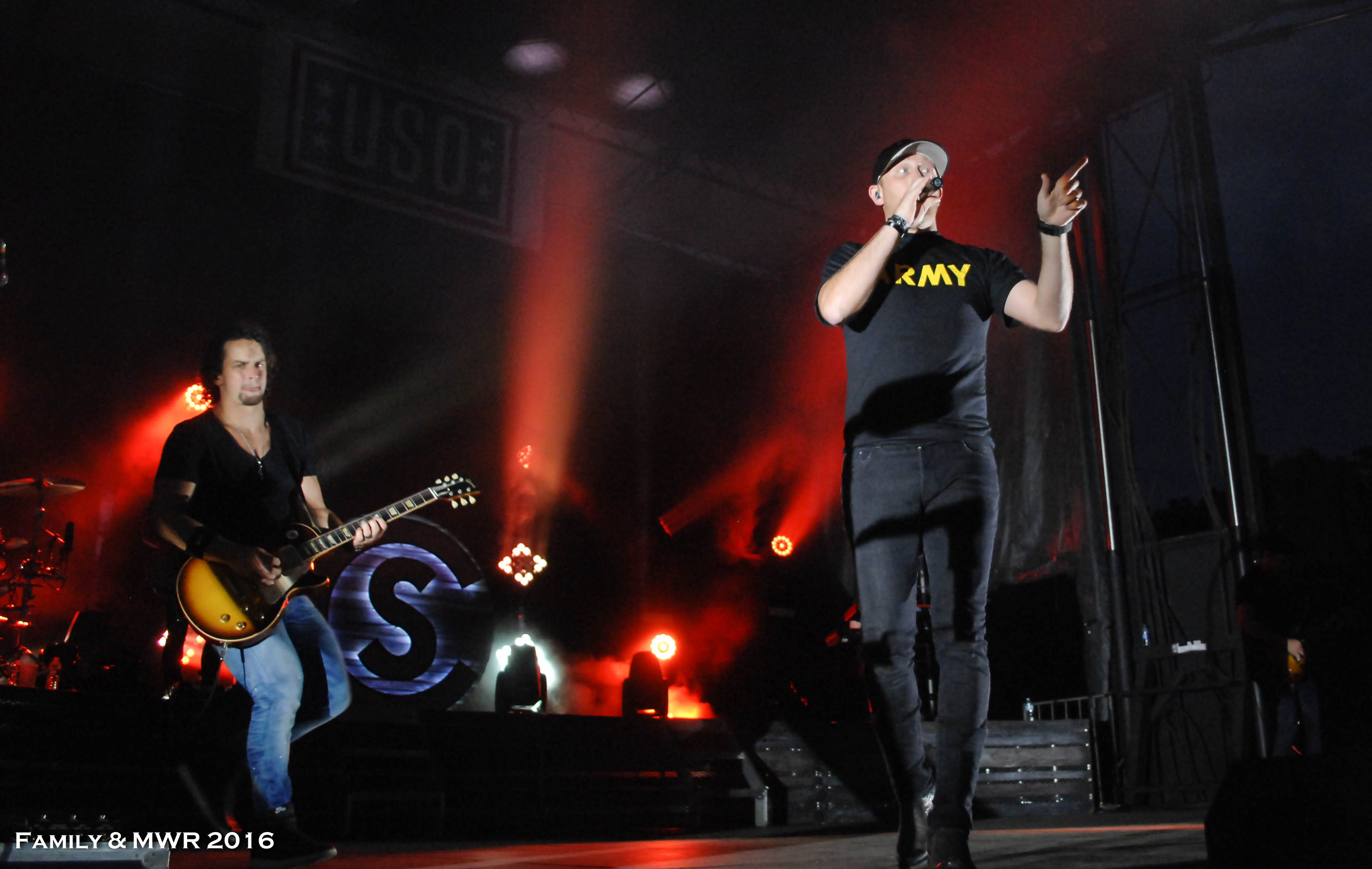The photograph captures Cole Swindell performing at what appears to be a USO concert. Positioned on the right side of the image, Swindell is decked out in black—wearing black shoes, black jeans, and a black shirt with "ARMY" emblazoned in yellow letters. A black baseball cap sits atop his head. He grips a microphone with his right hand, singing or speaking, while his left hand points outwards towards the audience. Adorning his wrists are a watch on his left and another band on his right.

To Swindell’s right stands a guitarist, dressed in a black t-shirt and blue jeans, playing a yellow and black guitar. The stage is bathed in red lights, with fog effects adding to the ambiance. The background features a drum set and a large 'S' logo. Near the top left of the image, a 'USO' sign is visible, hinting that this might be a USO show. Additionally, in the bottom left corner, the text "Family and MWR 2016" is displayed, further suggesting the event's context and date.